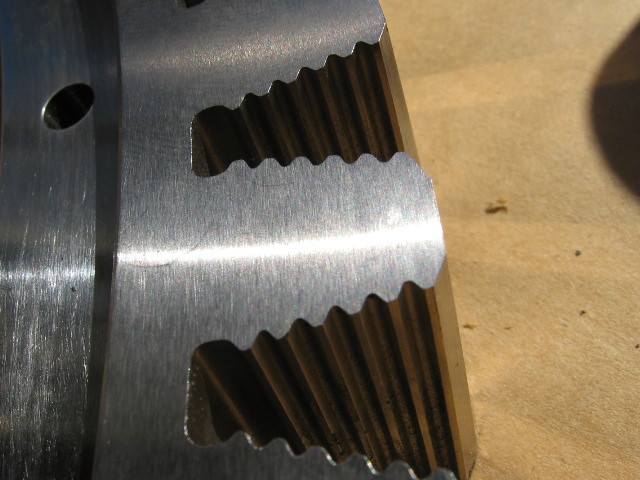This close-up photograph showcases the edge of a highly polished and milled silver metal object, likely a gear from a lathe. The gear features deep, striated teeth with vertical edges, which appear to be engraved and are prominent in the image. Two large, round holes or indents with a brownish, rusted tinge—likely due to extensive use—are positioned side-by-side on the gear's surface. The gear, partially visible and curved on the left, rests on what appears to be a light brown concrete ground, with a view of part of a wooden table or workbench to the right. The detailed gear teeth structure, combined with the worn internal parts, suggests this lathe gear has seen significant operational time in shaping either metal or wood objects.